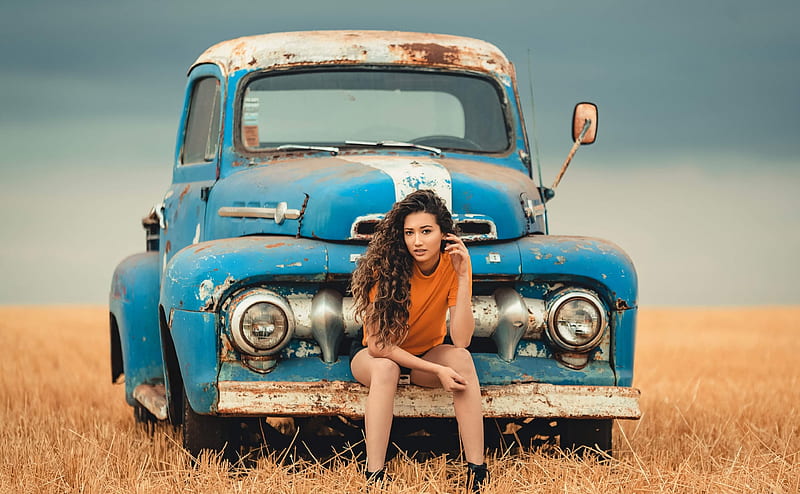In this evocative photograph, a young woman with long, curly brown hair sits confidently on the front bumper of a weathered 1940s blue truck, accented by rusty white trim and distinctive oversized wheel wells. Her outfit, more reminiscent of city life, consists of a short-sleeved orange shirt, very short black shorts, black ankle boots, and black socks. She strikes a pose with her right hand resting on her knee and her left elbow propped up, gazing with a model-like intensity at the camera. The scene unfolds against a flat, beige-brown field of what resembles mowed hay, under an ominous gray sky that deepens the nostalgic atmosphere. The old truck, possibly a Ford, with its large rusted-through patches and timeworn allure, enhances the rustic charm of the image.